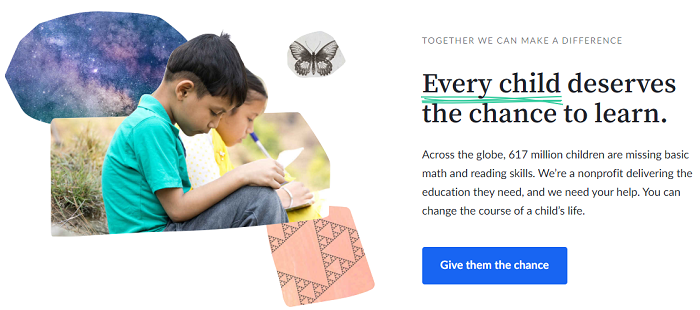The image features a white page filled with essential information about an educational nonprofit organization. The headline reads, "Together We Can Make a Difference," emphasizing the collaborative effort needed to address the issue at hand. Below it, a statement declares, "Every child deserves the chance to learn," underscoring the organization's mission. The page highlights a staggering statistic: "Across the globe, 617 million children are missing basic math and reading skills." This alarming figure sets the stage for the nonprofit's purpose—providing crucial educational resources to children worldwide. The page implores viewers for support with the message: "We are a nonprofit delivering the education they need and we need your help. You can change the course of a child's life. Give them the chance." 

An interactive element is present, likely a hyperlink labeled "Give them the chance," which suggests it may redirect users to a donation page for the nonprofit.

On the left side of the page, there is a poignant photograph of two young children, a boy and a girl, sitting on the ground. They are intently focused on writing on a piece of paper, symbolizing the thirst for knowledge that the organization aims to quench through its educational initiatives.